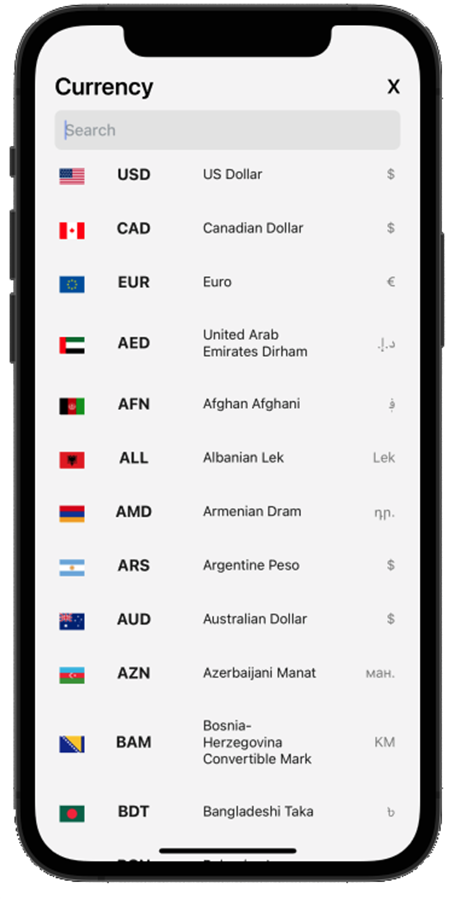In this image, prominently displayed at the top left corner is the word "Currency" in bold black text. Directly beneath this, there is a search bar with the word "search" in light gray text on the far left inside the bar. Below the search bar, a list of various currency names and their respective flags is presented. 

Starting from the top, the list includes the short names for each currency accompanied by their national flags on the immediate left. The list in descending order includes:

1. USD (U.S. Dollar)
2. CAD (Canadian Dollar)
3. EUR (Euro)
4. AED (United Arab Emirates Dirham)
5. AFN (Afghan Afghani)
6. ALL (Albanian Lek)
7. AMD (Armenian Dram)
8. ARS (Argentine Peso)
9. AUD (Australian Dollar)
10. AZN (Azerbaijani Manat)
11. BAM (Bosnian Convertible Mark)
12. BDT (Bangladeshi Taka)

Each currency abbreviation is followed by the full currency name written to the right. Additionally, the respective currency symbols are situated to the far right of each currency name, providing a comprehensive overview of the various international currencies.